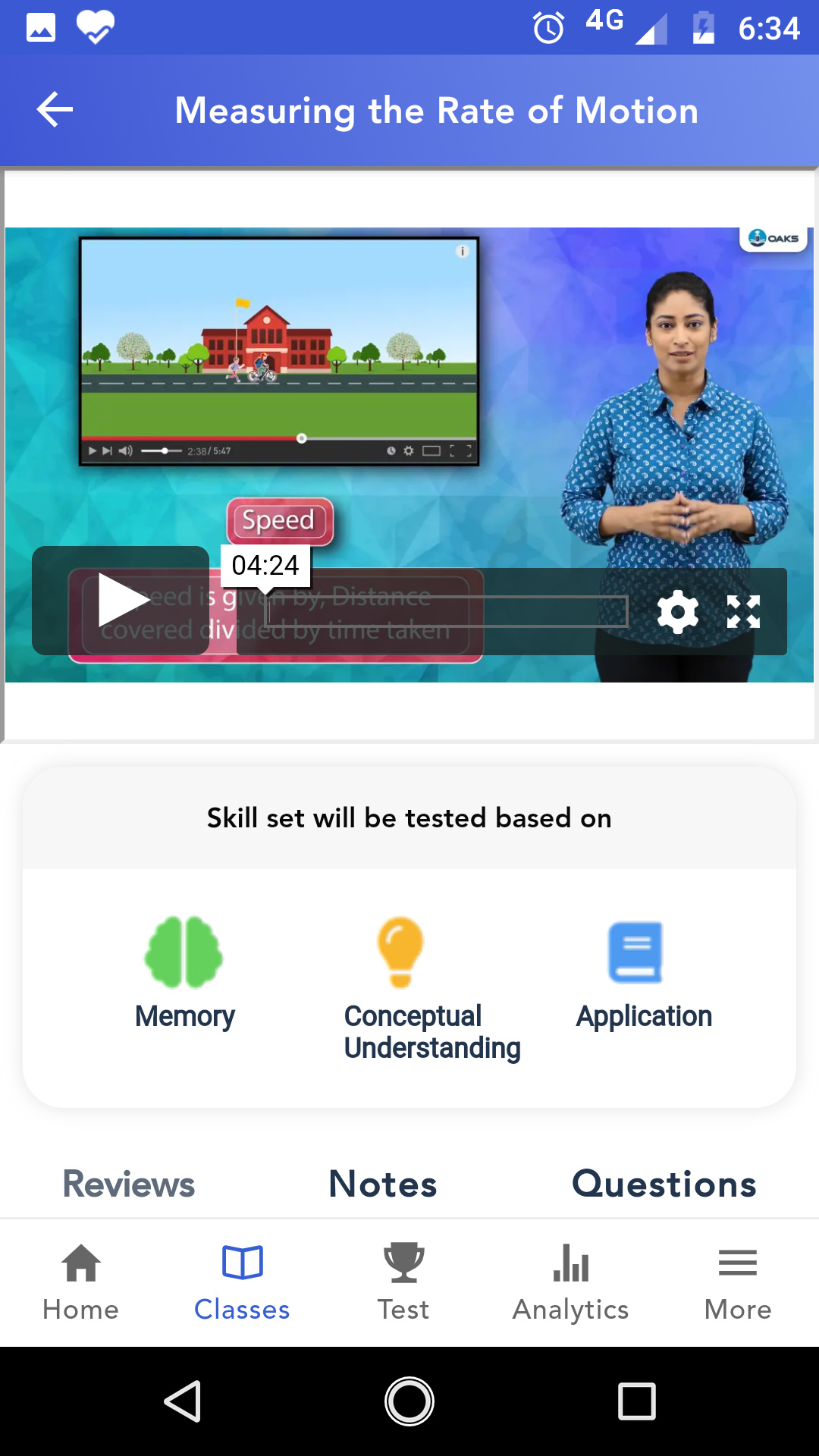The image is a cell phone screenshot featuring a user interface with multiple sections and vibrant colors. At the top, there is a purple bar with white cell phone icons indicating signal strength, battery life, and other standard notifications. Directly below is a lighter purple horizontal rectangle, with a gradient that transitions from dark on the left to light on the right. On the left side of this bar is a white, left-pointing arrow, and centrally placed in white text, it reads "Measuring the Rate of Motion."

Beneath this, a horizontal white rectangle spans across the screen, serving as a divider. Below the divider is a video player embedded within a colorful background gradient of purple, blue, and green. The top left of the video player displays a building on its screen, and to the right of the screen stands a woman. The bottom of the video player features a black play button, a progress bar, and icons for settings and full-screen view.

There is a strip of white immediately below the video player, followed by a light gray rectangle. Within this gray rectangle, dark gray text, centered at the top, reads "Skill Set Will Be Tested Based On." Lower down is a white horizontal bar containing three icons: "Memory," "Conceptual Understanding," and "Application," symbolizing different skill areas to be assessed.

Beneath this section, there are three options in black text: "Reviews" on the left, "Notes" centered, and "Questions" all the way to the right, each possibly representing different interactive features or sections related to the content.